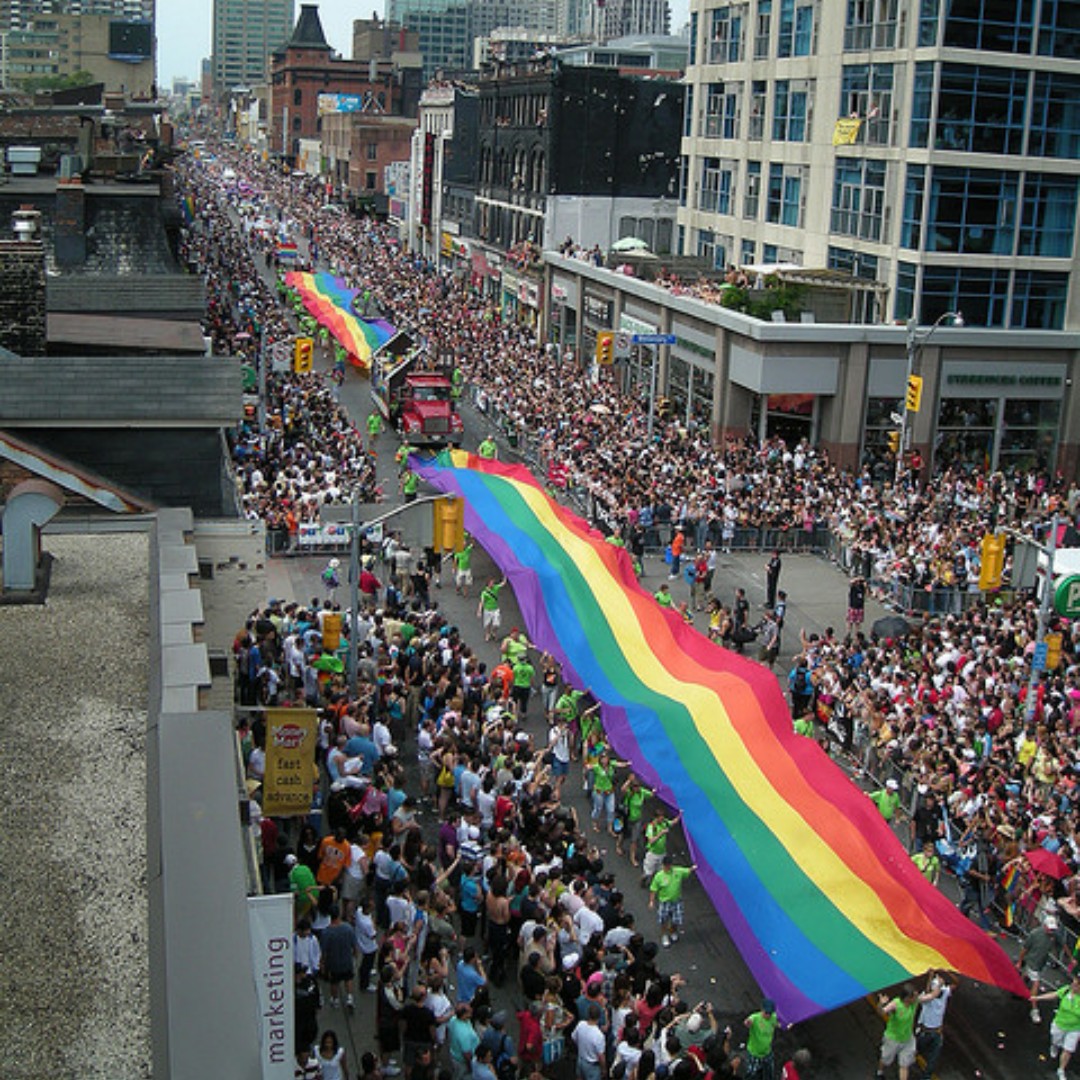The image captures a lively gay pride parade taking place in a bustling metropolitan city. Viewed from an elevated perspective, the shot looks down on a main street flanked by towering skyscrapers, with the parade spanning from the bottom left to the top right of the photo. Dozens of spectators line both sides of the street, illustrating the sizable turnout for the event. In the foreground, a group of people are seen carrying a very long rainbow flag, approximately half a block in length. Just behind this banner, a red semi-truck hauls what appears to be a small house. Further down the street, another large rainbow flag is held aloft by participants, followed by a procession of more vehicles and a vibrant sea of attendees, all donned in colorful attire. The festive and inclusive atmosphere of the parade is vividly captured, with rich details highlighting the unity and diversity of the celebration.